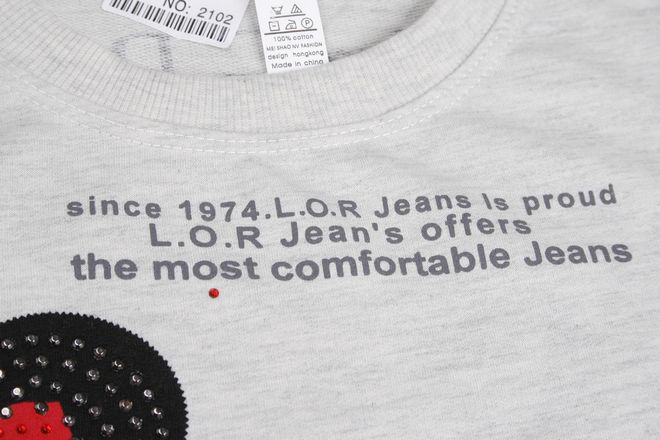The image is an extreme close-up of a shirt, focusing on the upper half with a crew collar. The shirt is light gray with a text print across the chest that reads, "Since 1974, LOR Jeans is proud, LOR Jeans offers the most comfortable jeans." Below the print, there's a small red dot under the "O" in "most." The shirt also features a decorative element in the lower left corner, consisting of a black circle with small black beads around its edge and a red segment inside, possibly part of a larger pattern. The label inside the shirt indicates it's made of 100% cotton and produced in China, with the number 2102 above a barcode. The shirt seems to have a thick material, resembling a sweater.